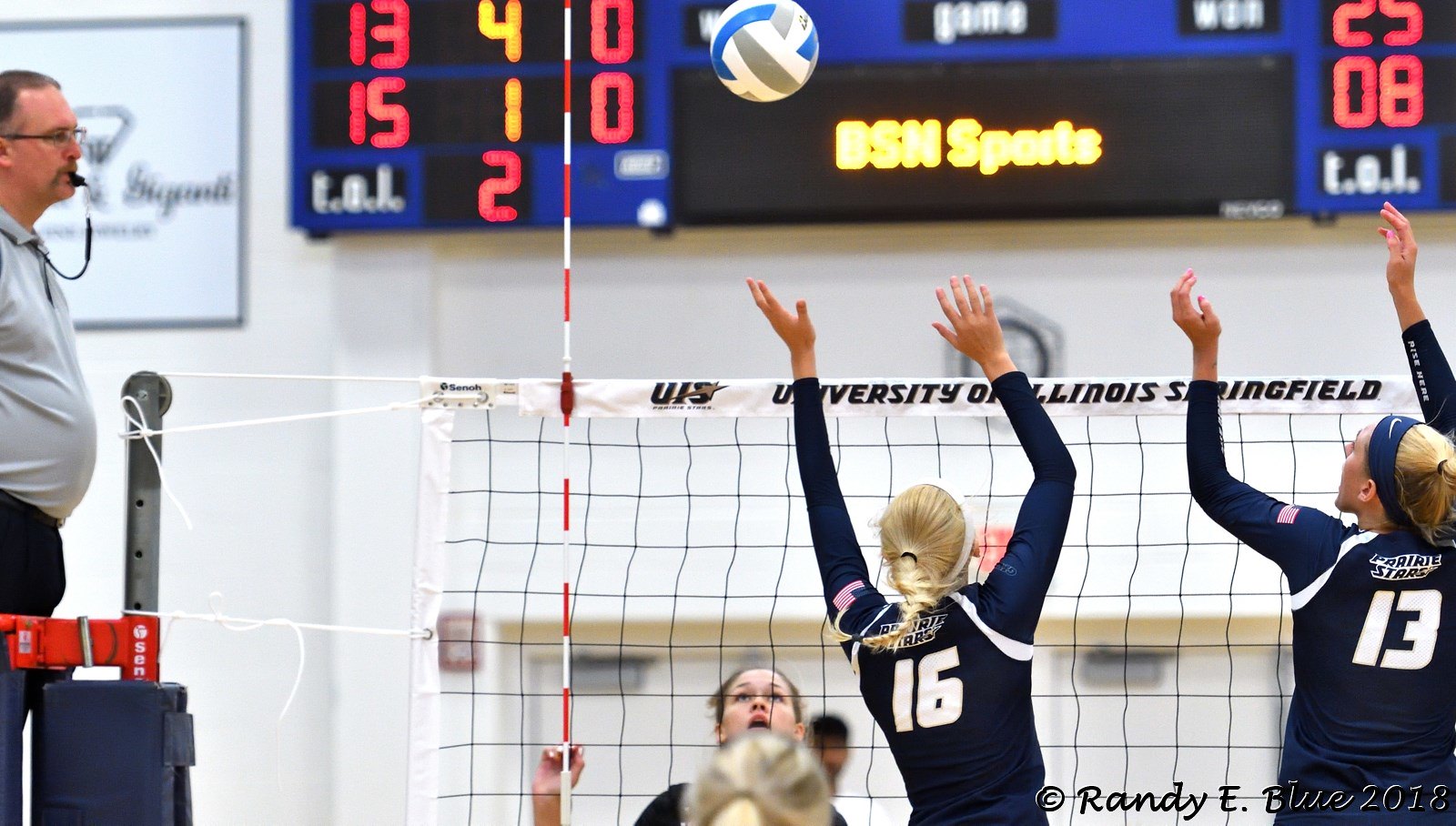This image captures an intense moment from a women's volleyball game inside a brightly-lit gymnasium with white walls. On the court, two players from the University of Illinois Springfield team, wearing matching blue long-sleeved jerseys with white shoulder stripes and numbers 16 and 13, are seen mid-air as they attempt to block the ball. Both players, who are blondes, have their arms extended upwards; the ball is positioned just above the left hand of the player with the number 16 jersey. On the other side of the net, another player is also partially reaching up, seemingly poised to intercept or having already struck the ball. The net prominently displays the text "University of Illinois Springfield" on its white strip. To the far left, a referee stands elevated on a small podium. He is wearing a white polo shirt, black pants, glasses, and has a whistle in his mouth. Above this action, a blue scoreboard with an electric backdrop showcases red numbers. The left side indicates a score of 13 and 15 below it, while the right side shows scores of 25 and 08. The middle of the scoreboard reads "BSN Sports" in yellow letters on a black background. The scene is vibrant and full of dynamic motion, emphasizing the athleticism and competitive spirit of the game.